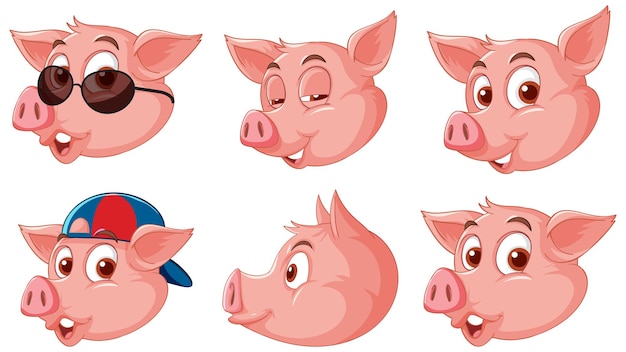This is a detailed, color illustration featuring six cartoon pig heads, arranged in two rows of three, all set against a white background. On the top left, a pig sports brown sunglasses with his mouth slightly open, showing his top teeth and his ears sticking straight out. Directly below him, another pig with the same expression and ears is wearing a backwards blue and red striped baseball cap. The pig in the top middle has his face slightly turned left, eyes squinting seductively, and a subtle smile. Beneath him, another pig with its profile facing left has wide-open eyes and upright ears, presenting a stark contrast. On the top right, a cheerful pig looks slightly to the left with brown eyes, showing his little teeth, one ear up, and the other to the side. Directly below this pig, another pig mirrors the top right's forward gaze, displaying similar ear positions, an open mouth revealing the top teeth, and an alert expression.